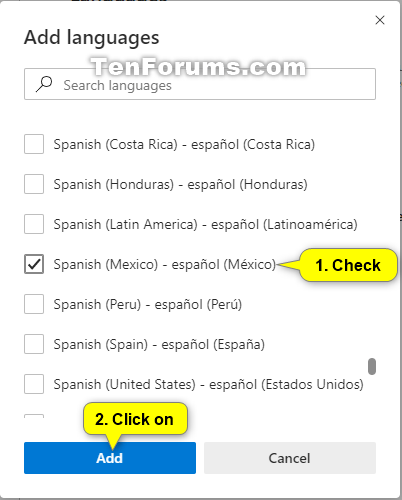The website interface displayed on the screen appears to have a rectangular shape with a black border encompassing the top, right, and bottom edges, while the left side remains border-free. 

In the upper right corner, there is a black "X" button. On the left side of the page, the header section includes the text "AdWord A" with a capital "A" followed by the word "Languages," both of which are highlighted in bold black text. Below this, there is a search bar consisting of a white rectangle outlined in black. Within this search bar, the placeholder text "Search Languages" is displayed in gray, accompanied by a black magnifying glass icon. Above the search bar, the website's title, "10forums.com," is prominently displayed in bold white text outlined in a grayish-black color.

On the main body of the webpage, there are multiple checkboxes aligned vertically on the left side, each framed by a gray outline with a white interior, allowing users to make selections. Adjacent to these checkboxes is a list of language options that users can choose from. The first option reads "Spanish (Costa Rica)" (Español (Costa Rica)), which is currently unchecked. The second option, "Spanish (Honduras)" (Español (Honduras)), is also unchecked. Similarly, the third option, "Spanish (Latin America)" (Español (Latino América)), remains unchecked. The fourth option, "Spanish (Mexico)" (Español (México)), differs as it is marked with a black check, indicating it is selected. Nearby, there is a yellow text box containing the number "1" in black.

Further down the list, additional unchecked language options are presented, including "Spanish (Peru)" (Español (Perú)), "Spanish (Spain)" (Español (España)), and "Spanish (United States)" (Español (Estados Unidos)).

At the bottom of the webpage, two prominent rectangular buttons are present. The first button is blue and labeled "Add," and it features an adjacent yellow text box with the black number "2" and the instruction "click one." The second button is gray and labeled "Cancel."